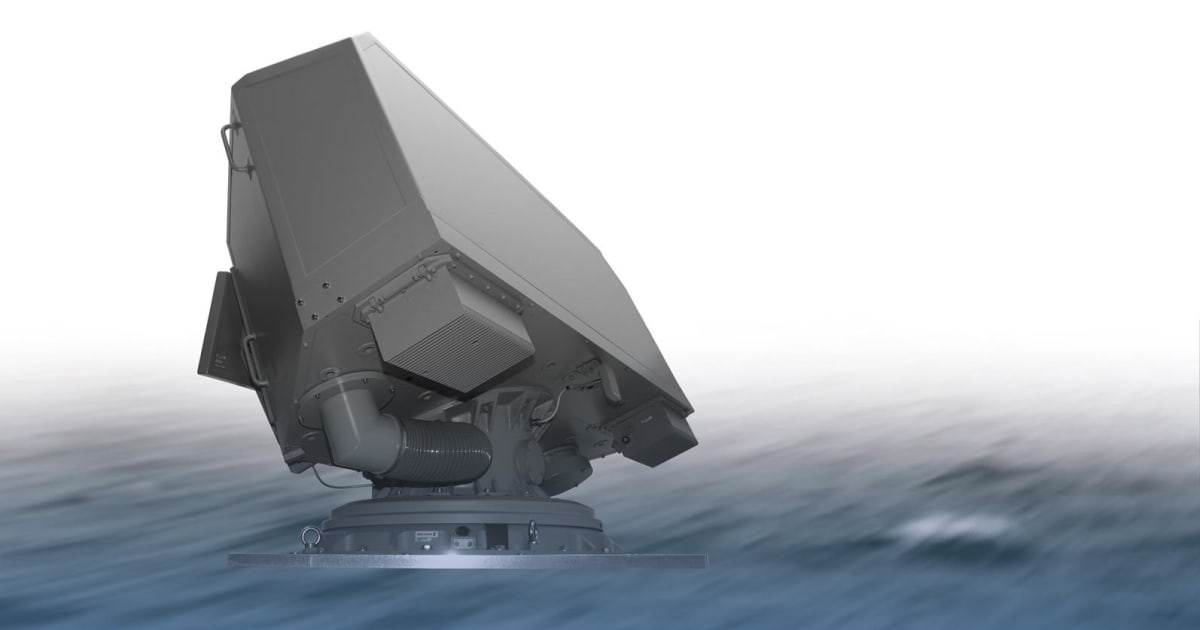The image appears to be an AI or Photoshop-generated scene, dominated by an off-white background that covers the top seven-eighths, while the bottom one-eighth features a bluish-gray hue reminiscent of water with faint diagonal wave patterns in dark gray and light black. Just left of center, a prominent metallic structure emerges as if rising from the water or clouds. The structure consists of a round base leading up to a narrower neck, topped by a larger, tilted rectangular box. This box, adorned with various smaller attachments, rivets, and bolting, includes tubes extending from its underside to the right. Metallic handles are visible on the corners of this assemblage, which exudes a slightly reflective sheen. Overall, the object resembles an extended-height Lego or an abstract buoy but also has elements suggesting it could be an electrical box or another type of industrial apparatus. The surreal placement and unclear context add to the image's enigmatic allure.